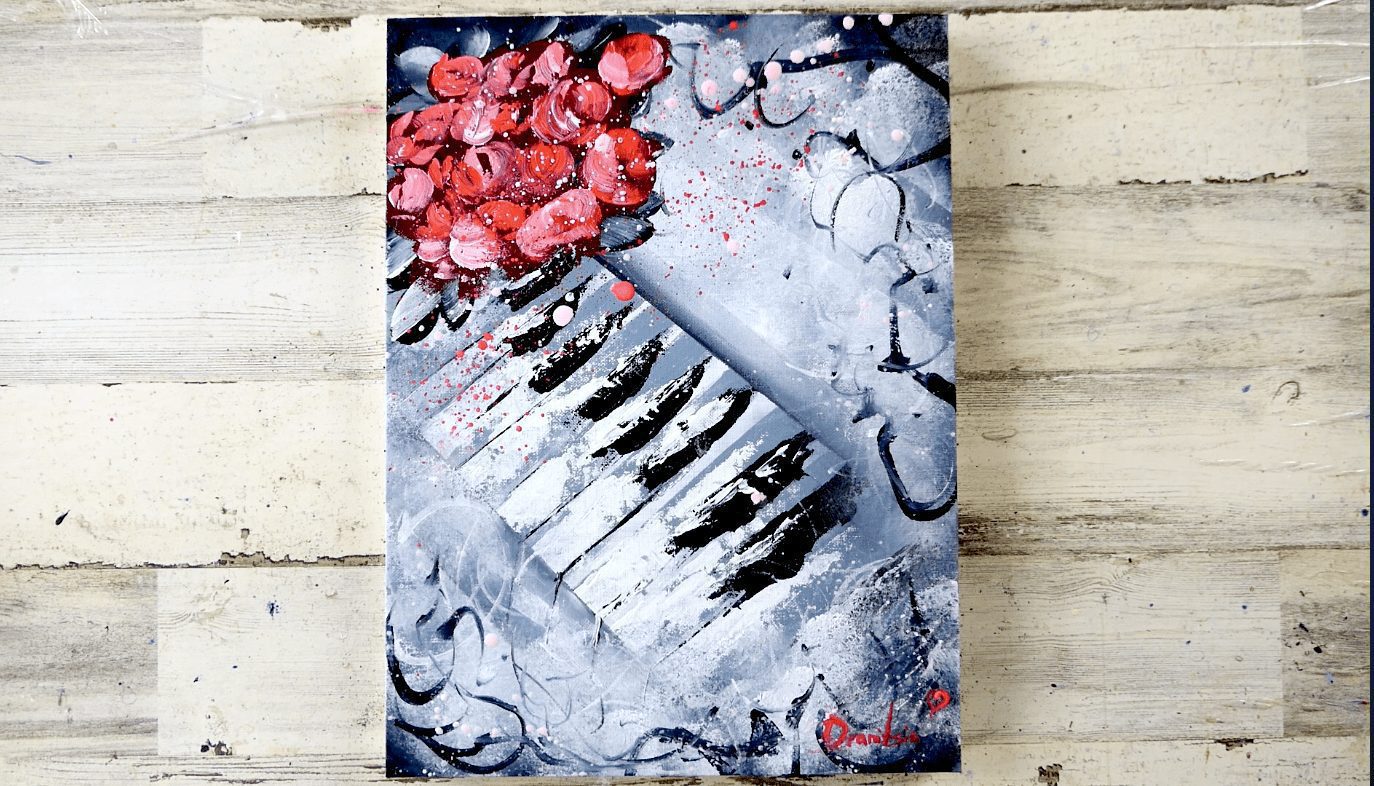The painting depicts a set of piano keys, rendered in a slightly chaotic and abstract style. The keys are mainly white bars with gray accents on the right or top and feature irregular, black streaks to indicate the black keys. Despite the abstract representation, there's a clear indication that these are piano keys. On the left side of the painting, clusters of red blobs, resembling flower petals, add a touch of vibrant color. The background appears predominantly grayscale, with swirling black patterns that might suggest branches or some form of natural growth, and the majority of the scene gives the impression of a wintery setting with the piano seemingly resting in snow. The lower right-hand corner of the painting includes a red signature. The entire artwork is mounted on beige-colored wooden planks, further suggesting a sense of rustic charm. The painting, primarily on canvas, conveys a sense of nature intermingling with music, as if the piano is part of a serene, yet slightly disordered, natural scene.